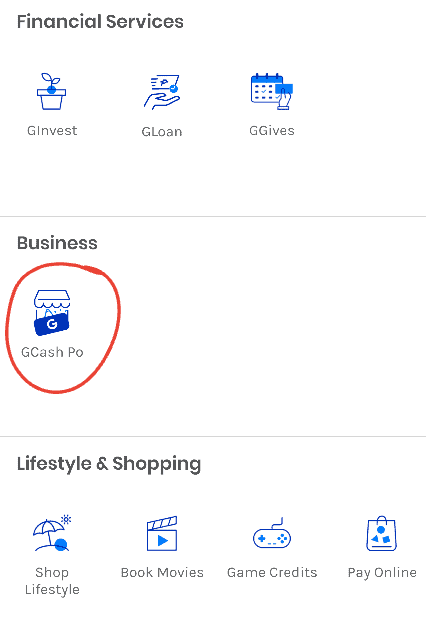This is a detailed descriptive caption for the image provided:

The image is a screenshot of an app with an all-white background. At the top left, in black text, it reads "Financial Services." Below this heading are three options: "G-Invest," "G-Loan," and "G-Gives." The "G-Invest" option is illustrated with a small potted flower, the "G-Loan" option features a hand and a check, and the "G-Gives" option is represented by a calendar. 

A gray horizontal line separates the "Financial Services" section from the next. The subsequent heading is "Business," under which there is one option: "G-Cash PO." This option has an image resembling a storefront with a dollar sign featuring the letter "G" on it. A red hand-drawn circle highlights the "G-Cash PO" option.

Another gray line divides the "Business" section from the next, which is labeled "Lifestyle & Shopping" in black text. This section features four options. The first option, "Shop Lifestyle," is on the left and is depicted with an illustration of a hill, an umbrella, a sun, and a blue dot. Next to it is "Book Movies," represented by a clapperboard used in film production. To the right of this, "Game Credits" is shown with a game controller above the text. The final option, "Pay Online," has an illustration of a shopping bag adorned with a circle, a square, and a triangle.